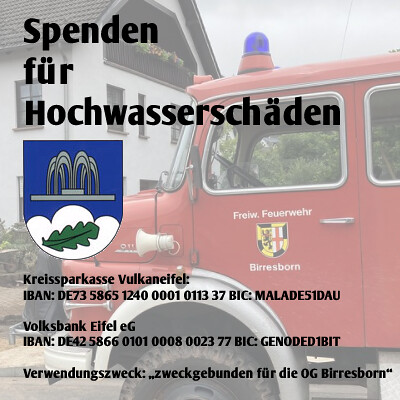In this daytime outdoor advertisement, we see a photographic image of a vintage red fire engine with distinctive features including a blue siren on top, a prominent white horn on the driver's side, and a black tire. The vehicle is parked in front of a picturesque white, two-story house with a gabled roof, a balcony adorned with flowers, and a window box. The scene is enriched with greenery visible through the truck's windows, adding a touch of natural beauty to the setting.

The fire truck's door bears an emblem featuring a St. George cross and flowers, alongside the text "Freiw. Feuerwehr Birresborn" with a silver handle—highlighting that it belongs to the volunteer fire department of Birresborn. 

Overlaying this image is foreign text promoting a cause: "Spenden für Hochwasserschäden" (translated as "Donations for Flood Damage"). This is accompanied by donation details and a logo depicting a fountain on top of a white cloud with a leaf embedded in it. Additional text includes banking details for donations, indicating the message's charitable nature. The visual combination of the fire truck and the house provides a nostalgic and community-focused backdrop to this important call for aid.